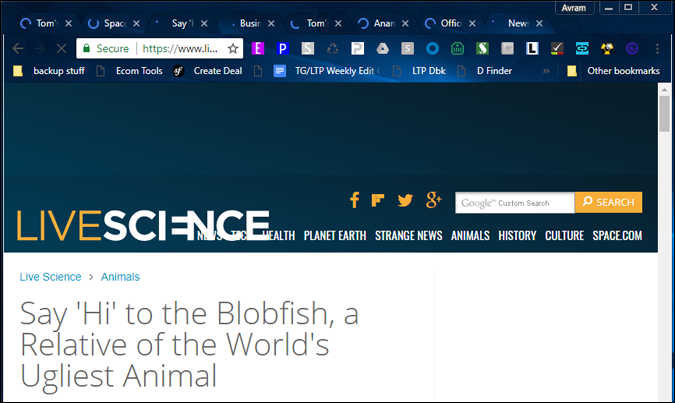A cluttered web browser window is displayed, featuring an article from a live science website with the headline, "Say Hi to the Blobfish, a Relative of the World's Ugliest Animal." The screen shows numerous tabs open, all appearing to be in the process of loading, possibly indicating issues with the internet connection. The website in question seems unfamiliar and unused by the viewer, adding an element of curiosity to the scene. The overall image captures the common modern-day scenario of navigating multiple online pages simultaneously, sometimes leading to connectivity challenges.